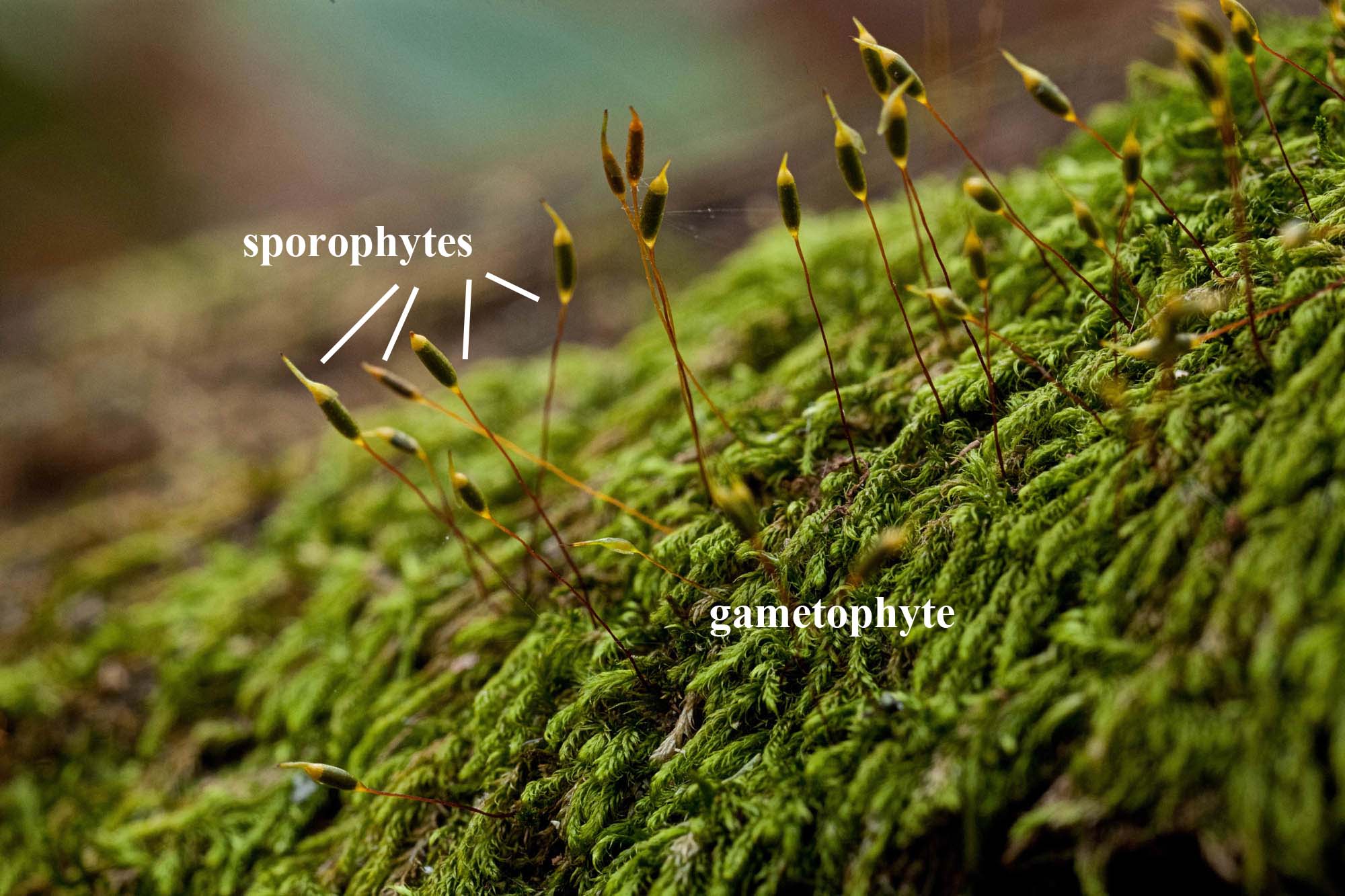This close-up, horizontally rectangular image captures intricate details of a green plant structure with labels for clarification. The blurred background, featuring greens, yellows, and reds, ensures focus on the foreground. Emerging from the dense, leafy fronds, slender stalks with tiny, pod-like structures resemble miniature cattails. The top left corner of the image includes the label "sporophytes" in white font, pointing to these protruding stalks. In the midst of the verdant foliage, the label "gametophyte" is also displayed in white, helping to identify the main body of greenery. The overall coloration of the image predominantly utilizes shades of green, with hints of yellow and dark tones accentuating the details.